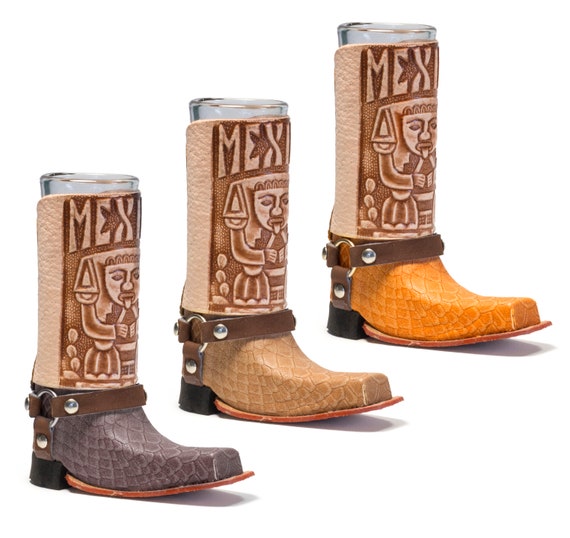This image features a set of three intricately designed souvenir boots, presumably from Mexico, each presented against a stark white background which heightens their visual prominence. All three boots share a consistent style, distinguished primarily by the color of the shoe portion. 

The boot on the left has a snakeskin-like texture with a dark purple hue and features a brown heel, a brown strap near the ankle, and a brown leather section extending up the leg, emblazoned with the letters "MEX" above a tiki-like face with its tongue out. Adding to its uniqueness, the very top of this boot seems to include a glass-like material. 

The middle boot mimics the left one in design, but the shoe part is a light tan color. This boot also has a brown heel and strap, with the same "MEX" inscription and tiki face on the leather upper portion.

The rightmost boot, also mirroring the overall design, showcases an orange-colored shoe part. It maintains the recurring features of a brown heel and strap, with the same "MEX" lettering and ancient tiki-like face on its leather upper portion, and a glass-like top accent present across all three boots.

Each boot demonstrates a harmonious blend of rustic charm and cultural artistry, encapsulating the essence of Mexican craftsmanship.